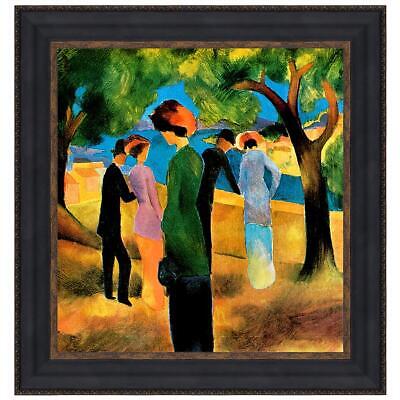This artwork, framed in an almost black dark brown wood frame with a lighter brown inner border, presents an abstract scene infused with early 1900s modernist influences. The color palette predominantly features greens, yellows, browns, and blues. The ground in the painting is depicted as a yellowing brown, while the sky is a soft baby blue. Standing in the center is a woman with red hair, wearing a green jacket over a black dress. She is slightly apart from two couples closer to the water's edge—both couples consisting of men in black suits with black hats, and women in long, simple dresses and sun hats. One woman wears a pink dress with a sun hat, while the other wears a lilac jacket over a blue dress. The figures are positioned on a brown grassy hill with bright green foliage on trees flanking the left and right sides of the image. The water at the center, possibly a bright blue river, features an island in the distance, and there are buildings seen at the bottom left of the hill. The overall scene emits a somber tone, ostensibly owing to the separateness of the central woman, creating a subtle contrast in the otherwise serene landscape.